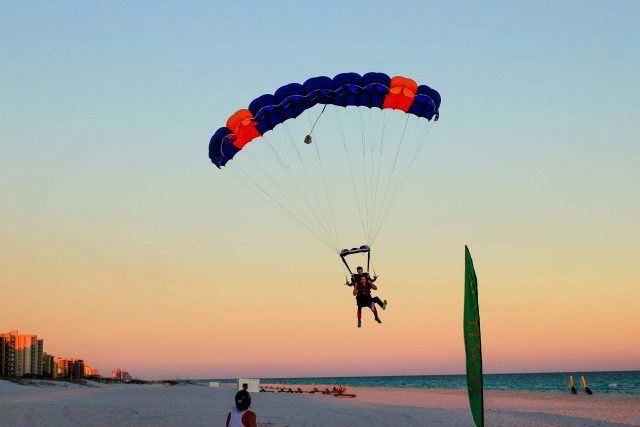In this detailed photograph captured at sunset, two people are paragliding above a serene beach landscape. The scene unfolds under a breathtaking dusk sky, which transitions from a deep blue at the top to soothing shades of peach, pink, and orange towards the horizon. The pair is securely harnessed to a vividly colored parachute, marked by dark navy blue with striking orange stripes on its edges. The parachute, featuring multiple channels, hovers gracefully above, brightly contrasting against the multicolored sky. Below them, the sandy beach stretches out smoothly, depicted in earthy brown hues, and the calming waters of the ocean shimmer in greenish-blue tones, reflecting the dwindling daylight.

The beach itself is dotted with elements of human presence; on the far left, a series of tall high-rise buildings stand vigil along the shore. An onlooker, partially cut off in the frame, watches in awe from the sand, adding a sense of scale to the hovering paragliders. In the scene, a green flag flutters in the land breeze, though its inscription remains indistinguishable. The absence of clouds accentuates the clarity and tranquility of the moment, encapsulating the serene yet exhilarating experience of paragliding at dusk over an idyllic seaside setting.